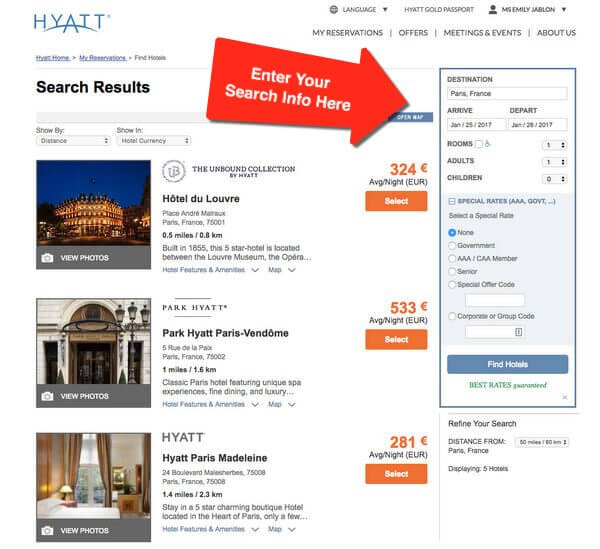This image is a detailed screenshot of the Hyatt website, showcasing a comprehensive interface for users to manage their reservations and explore hotel options. At the top left, the classic Hyatt logo is prominently displayed, while the top right corner includes navigation options such as language settings, Hyatt Gold Passport access, and a personalized greeting for the logged-in user, Ms. Emily Jablon. The menu bar offers a variety of options including 'My Reservations', 'Meetings and Events', and 'About Us'.

On the left side of the screenshot, search results are displayed, featuring three hotel options based on the entered criteria. Each hotel option includes a photo, a brief description, distance from the entered location, pricing details, and a selection button for more information.

The right side of the screen is highlighted, drawing attention to a blue-highlighted search box marked by a giant red arrow. This section invites users to input search details such as destination, arrival and departure dates, the number of rooms, the number of adults and children, special rate codes, and offers the ability to refine the search.

The overall layout and design of the website suggest it may be an example site intended to help users become familiar with the search and reservation process, providing clear, step-by-step guidance to easily navigate and select accommodations.